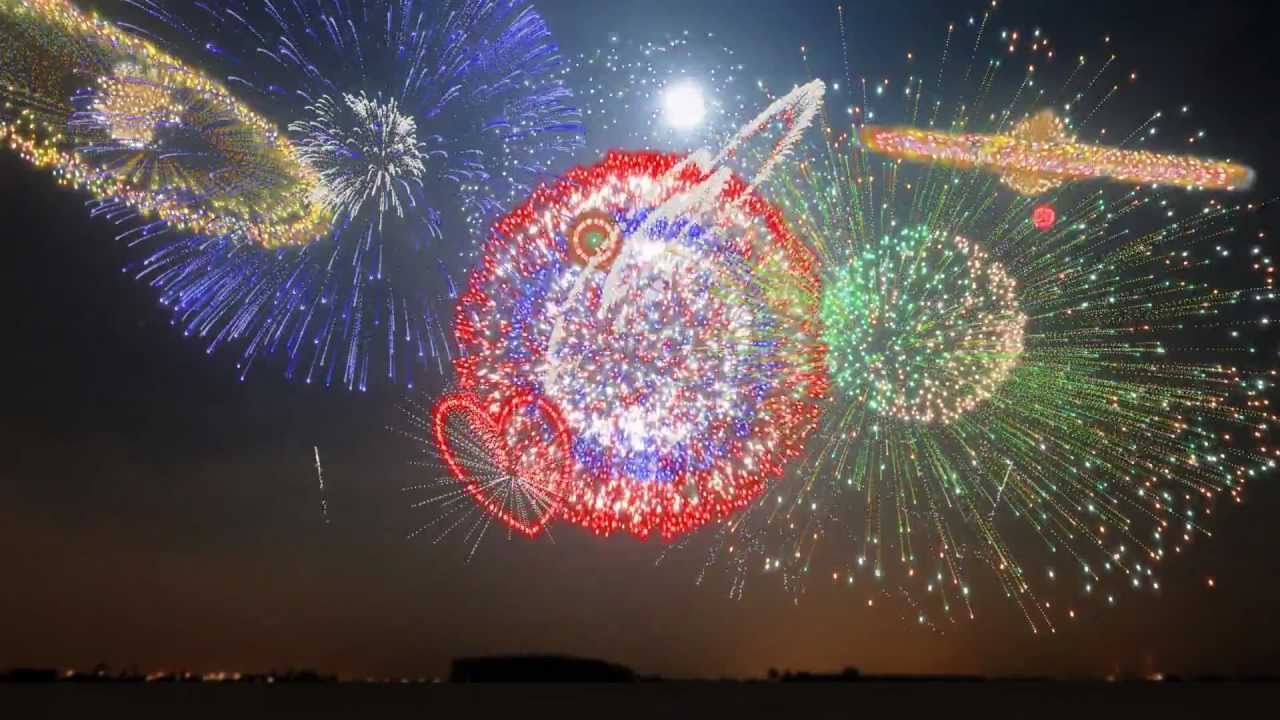Against the backdrop of a black night sky, this vibrant photograph captures a dazzling array of fireworks exploding over a silhouetted city skyline. To the top left, a distinctive yellow firework with a ring and a central circle catches the eye, complemented by a blue firework bursting in a classic starry pattern. Dominating the middle of the scene is a stunning red heart-shaped firework, alongside a larger red firework fringed with red, white, and blue hues. To its right, a green and yellow firework radiates outward like a ball, while a yellow firework resembling Saturn graces the top right corner. The skyline below is dark, allowing the multitude of colors—yellow, blue, red, white, green, and gold—to illuminate the sky spectacularly, with small yellow lights adding a shimmering effect. Each firework's explosion contributes to a collective brilliance, painting the night with vibrant, breathtaking patterns.